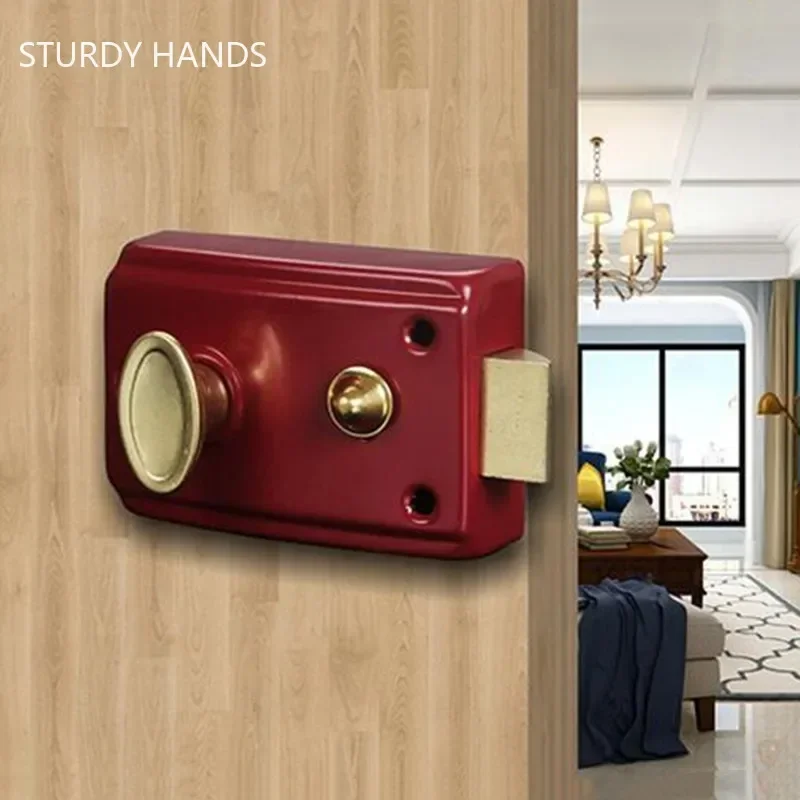The square image primarily features a thick wooden sliding door on the left side, with a detailed red rectangular device, potentially a lock or alarm, affixed at the center of the door. The device includes an oval gold knob on the left, a smaller gold cone-shaped protrusion to the right, two small cut-out holes, and a gold triangular handle at the bottom. In the upper left corner of the image, "STURDY HANDS" is written in all-caps white letters. The door is in a light wood shade and slightly ajar, showing its thickness. The right side of the image reveals a glimpse into a living room. There is a white-cloth ottoman with a navy blanket draped over it, a patterned beige area rug with a brown trim, and a light gray marble floor. Further into the room, there is a brown wooden table adorned with a white vase holding green plants, several white books stacked beside it, and a classy chandelier hanging from the white ceiling. Large windows overlook a cityscape in the background, completing the scene.